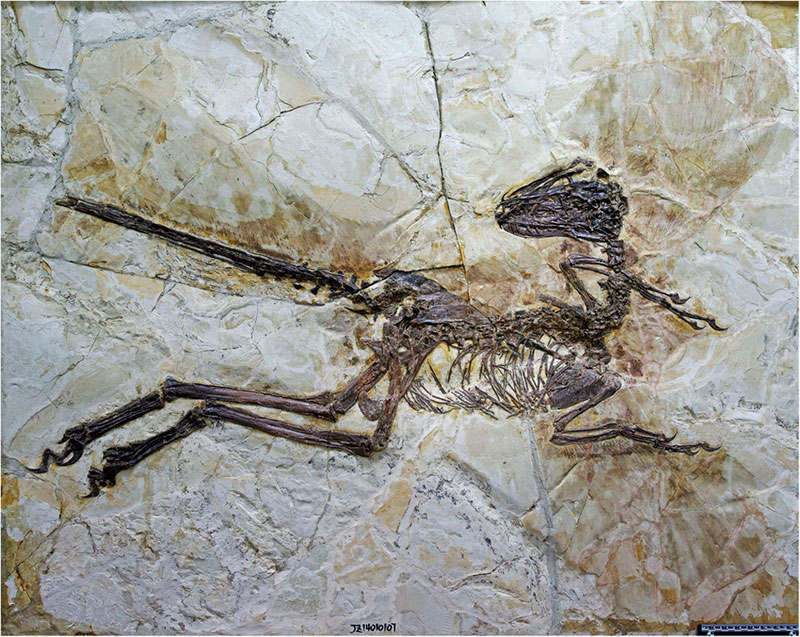The photograph showcases a close-up of a fossilized creature embedded in a lighter-colored slab of rock, ranging from light brown to white, providing a stark contrast to the dark brown to black bones. This well-preserved specimen features a thin, triangular head that is bird-like, turned backwards over its spine and body, which are angled to the right. The fossil highlights a long tail extending towards the left-hand side, almost the length of its entire body, with visible vertebrae. Noticeably, it has two very long, bent legs comprised of three distinct bones each, ending in feet or claws, suggesting mobility. The forearms, possibly wings, and a ribcage are shorter and folded up against its body, with some potential feather imprints visible in the rock. Additionally, there is a symbol and the number 14010107 inscribed on the lower section of the stone.